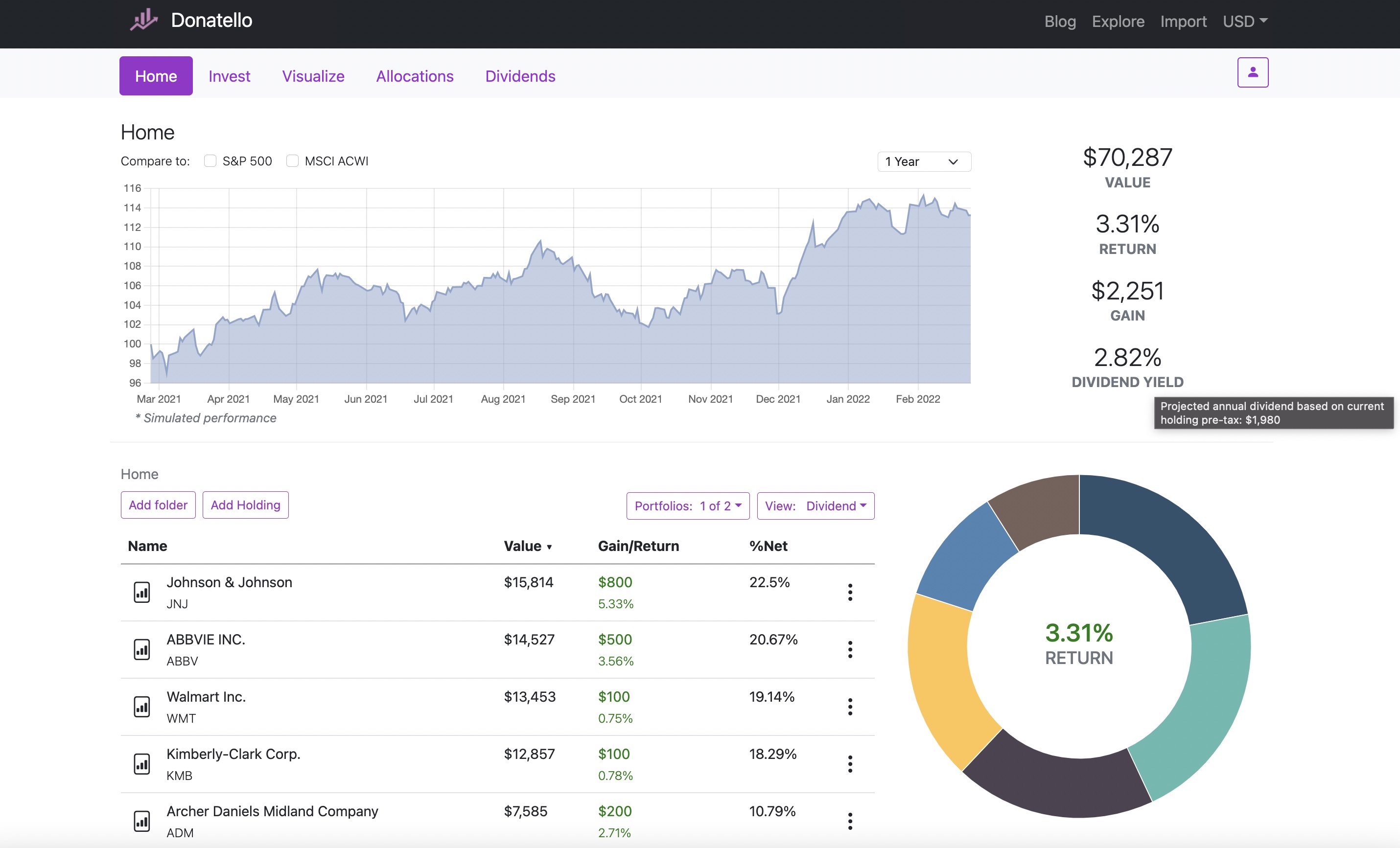The image is a detailed stock analysis page for a stock called Donatello. At the top of the interface, the "Home" section is highlighted, with options for "Invest," "Visualize," "Allocations," and "Dividends" listed beside it. Spanning the top part of the page is a graph that depicts the stock's performance over time. The y-axis of the graph has numerical markers ranging from 96 to 116, while the x-axis lists monthly intervals starting from March 2021 and extending to February 2022.

Above the graph, there is a dropdown menu labeled "One Year," indicating the timeframe of the data. Below this, a note reads "Simulated Performance". Further down the page, there are options labeled "Home," "Add Folder," and "Add Holding". The page details individual stock entries, starting with "Johnson & Johnson" valued at $15,814, and listing others such as Walmart and Kimberly Clark, each accompanied by their value, gain/return, and percentage net categories.

On the right side of the page, key financial metrics are summarized: a portfolio value of $70,287, a return of 3.31%, a gain of $2,251, and a dividend yield of 2.82%. At the bottom right-hand side, a multi-colored pie chart visualizes these figures. The chart includes segments in various colors—yellow, blue, olive, light blue, and black. At the center of the pie chart, the return percentage of 3.31% is displayed prominently.